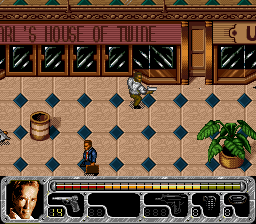This is a 2D video game screenshot, likely depicting an exterior courtyard area in front of a building named "RL's House of Twine." The courtyard features a pattern of dark blue diamond-shaped tiles set within larger brown tiles. A prominent green plant is visible on the right side of the scene. 

Two characters are present: the main character, standing directly in front of the twine shop, is equipped with a metal suit of armor and brown pants. The character's inventory display at the bottom left of the screen indicates several guns and possible ammunition slots. Another character, possibly a businessman, is visible walking towards the left, carrying a brown suitcase and dressed in a blue suit.

Additional interface elements include a health bar and the main character’s portrait, suggesting this is a standard RPG or adventure game interface. The partial visibility of a name at the top hints at potential cut-off naming due to the screenshot's aspect ratio.